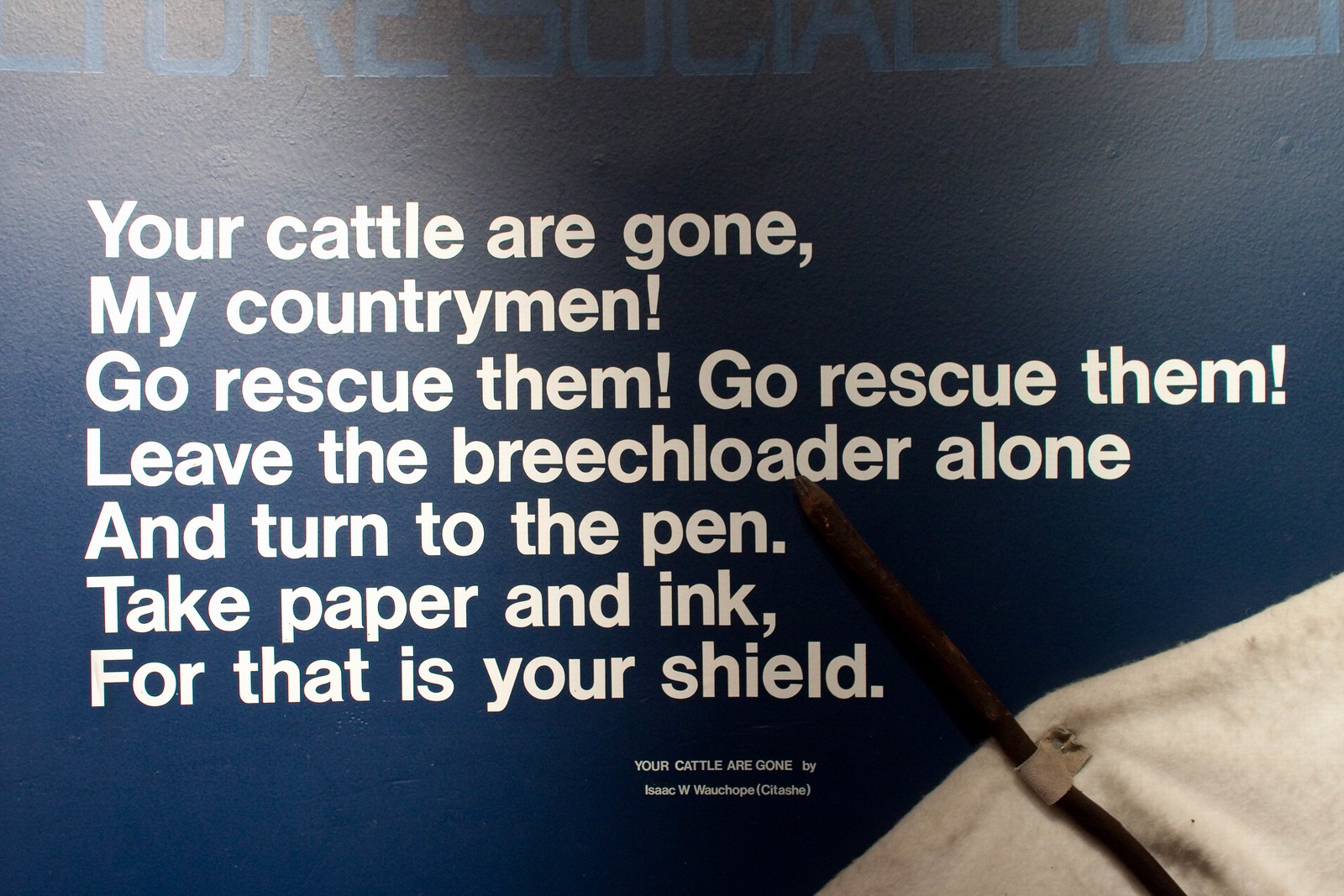On a navy blue background, partially obscured letters appear at the top of the image, and the bottom right corner shows a white cloth with what appears to be a branch or stick pinned to it. The central text, in large white print, delivers a rousing call to action, reading: "Your cattle are gone, my countrymen! Go rescue them! Go rescue them! Leave the breech loader alone, and turn to the pen. Take paper and ink, for that is your shield." Below this exhortation, a smaller print attribution reads, "Your cattle are gone by Isaac Wauchope (c-i-t-a-s-h-e)." The image evokes a sense of urgency, urging the reader to abandon arms in favor of written word, encapsulating the adage that the pen is mightier than the sword. The overall impression is of a pamphlet or poster, designed to inspire and motivate towards nonviolent action and reclamation of property.